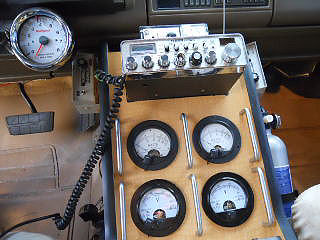This image showcases the control panel of a vehicle, likely a specialized utility or commercial truck. On the left side, the gas and brake pedals are clearly visible. Above these pedals, the dashboard features a tachometer or speedometer. Centrally located, a box with four distinct gauges is mounted, though the specific readings are blurred out. Above this box sits a radio, potentially a CB radio, with a coiled telephone cord extending from its left side towards the driver's area. On the far left of the control panel, a fire extinguisher is mounted for safety. In the lower right corner of the image, part of the passenger seat is visible. The interior features brown floor mats and a brown dashboard. Flanking the central gauge box, there are twelve small silver metal handles or levers, six on each side. The scene suggests a vehicle equipped for specialized tasks, with a focus on operational control and safety features.